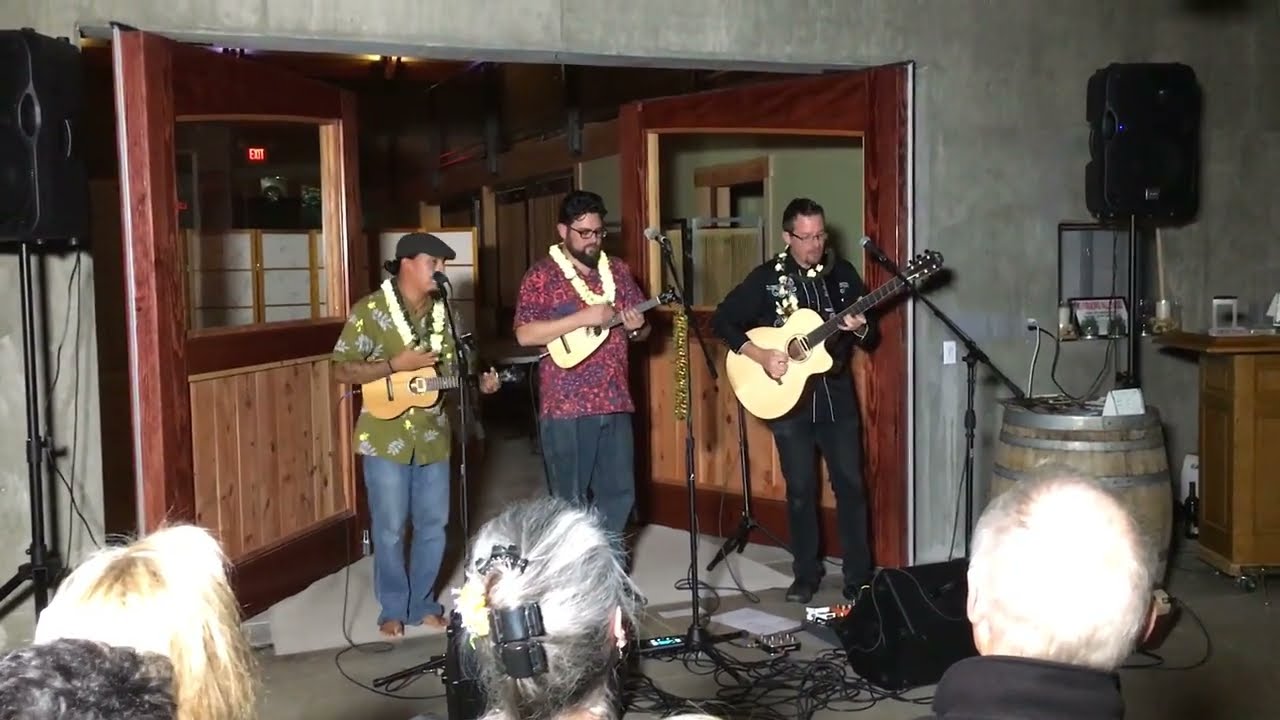In a cozy studio or concert hall, the photograph captures three Caucasian men serenading a small audience of four with their musical talents. Standing before partially open wooden doors, the band members each sing into their own microphones. On the right, a man in a black shirt and white lei strums an acoustic guitar. The middle musician, sporting a beard, mustache, glasses, and a purple shirt with a white lei, deftly plays a mandolin. To the left, the third member, donned in a green shirt, blue jeans, a scally cap, and a white lei, plucks a ukulele. The intimate audience, consisting of two women (one with a clip-on bow) and a man, closely watches the performance. Behind the musicians, wooden panels and a set of speakers frame the scene. Further to the right, a bar setup with a rolling cart, a barrel, and a mirror can be seen under a gray wall. The ambiance is one of heartfelt connection, as the small crowd is engrossed by the melodic ensemble.